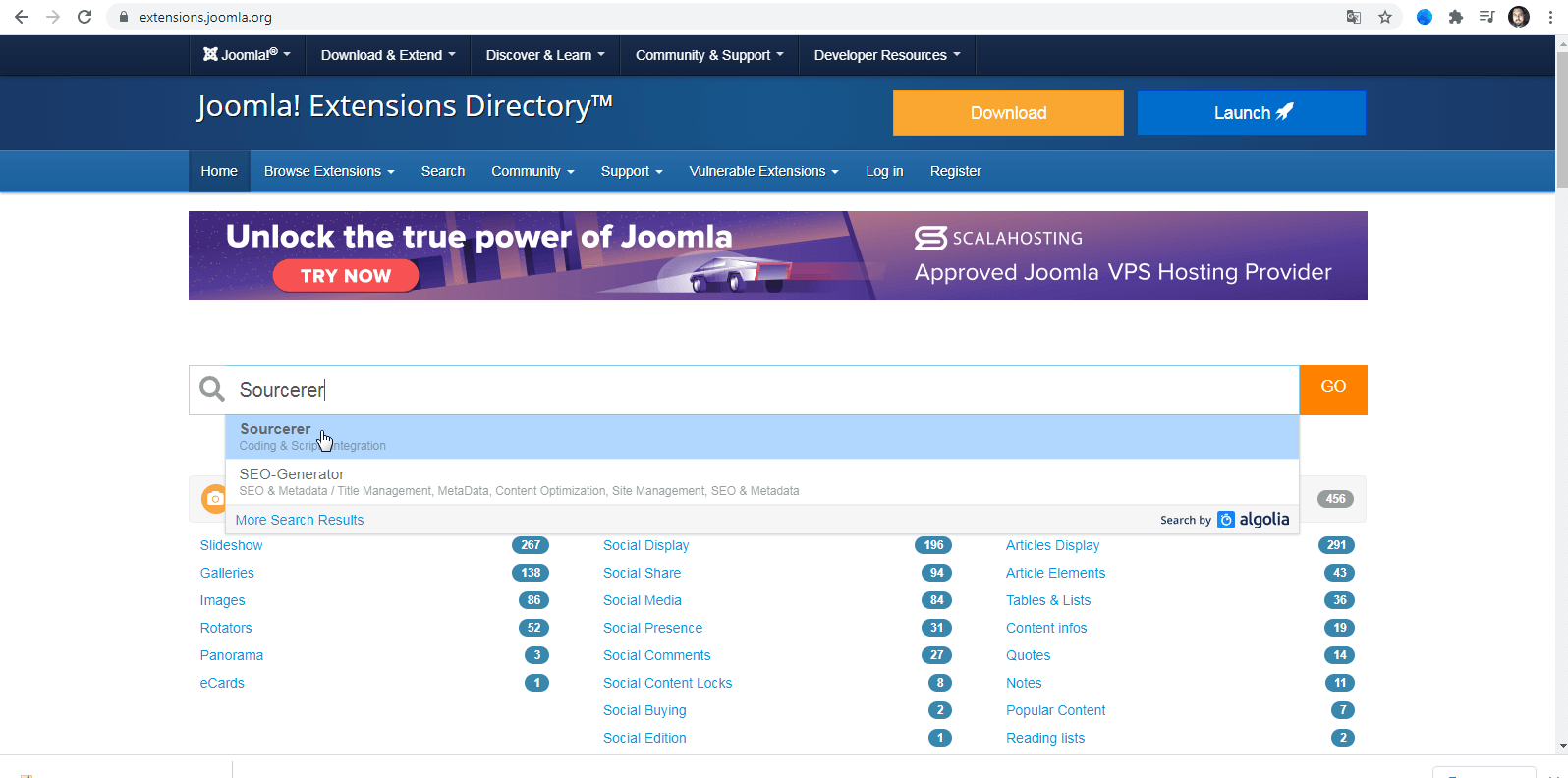The homepage of the Joomla! Extensions Directory is displayed prominently. At the top, a thin black bar showcases various logos, lending a professional touch. The main header, "Top Joomla! Extensions Directory," is presented in blue text with a subtle light blue gradient effect, drawing attention. Below this, a search bar invites users to "source server," accompanied by an orange "Go" button for quick navigation. Scattered across the page are numerous teal, pill-shaped icons, each representing different file names, although the text is too small to discern. Dominating the center is a vibrant purple banner ad with the empowering message, "Unlock the power of Joomla!"